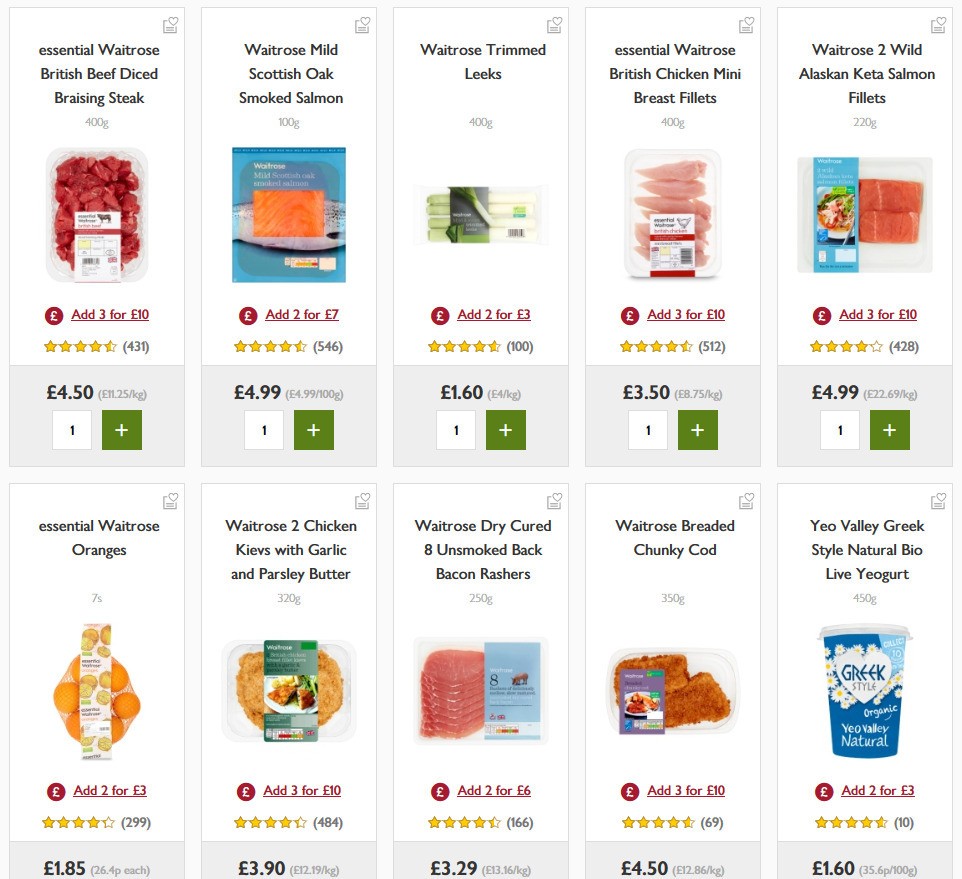This image is a detailed screenshot from a UK-based grocery website, featuring a clean white background and two rows of product listings, each displaying five items. 

**Top Row (Left to Right):**
1. **British Beef Diced Braising Steak** – Displayed in a white tray.
2. **Scottish Oak Smoked Salmon** – Showcased as a fillet.
3. **Leeks** – Shown as several stalks, visually similar to large green onions.
4. **British Chicken Mini Breast Fillets** – Contained within a tray.
5. **Alaskan Keta Salmon Fillets** – Packaged fillets with a reddish color.

**Bottom Row (Left to Right):**
1. **Oranges** – Presented in a mesh bag.
2. **Chicken Kievs with Garlic and Parsley Butter** – A prepared food item.
3. **Unsmoked Back Bacon Rashers** – Displayed in a transparent package.
4. **Waitrose Breaded Chunky Cod** – Packaged in a plastic tray.
5. **Yeo Valley Greek Style Natural Bio Live Yogurt** – Packaged in a blue container.

Each product includes a picture and name, with prices listed in pounds sterling, indicating the UK origin of the website. The selection mainly consists of diverse seafood and meat products.